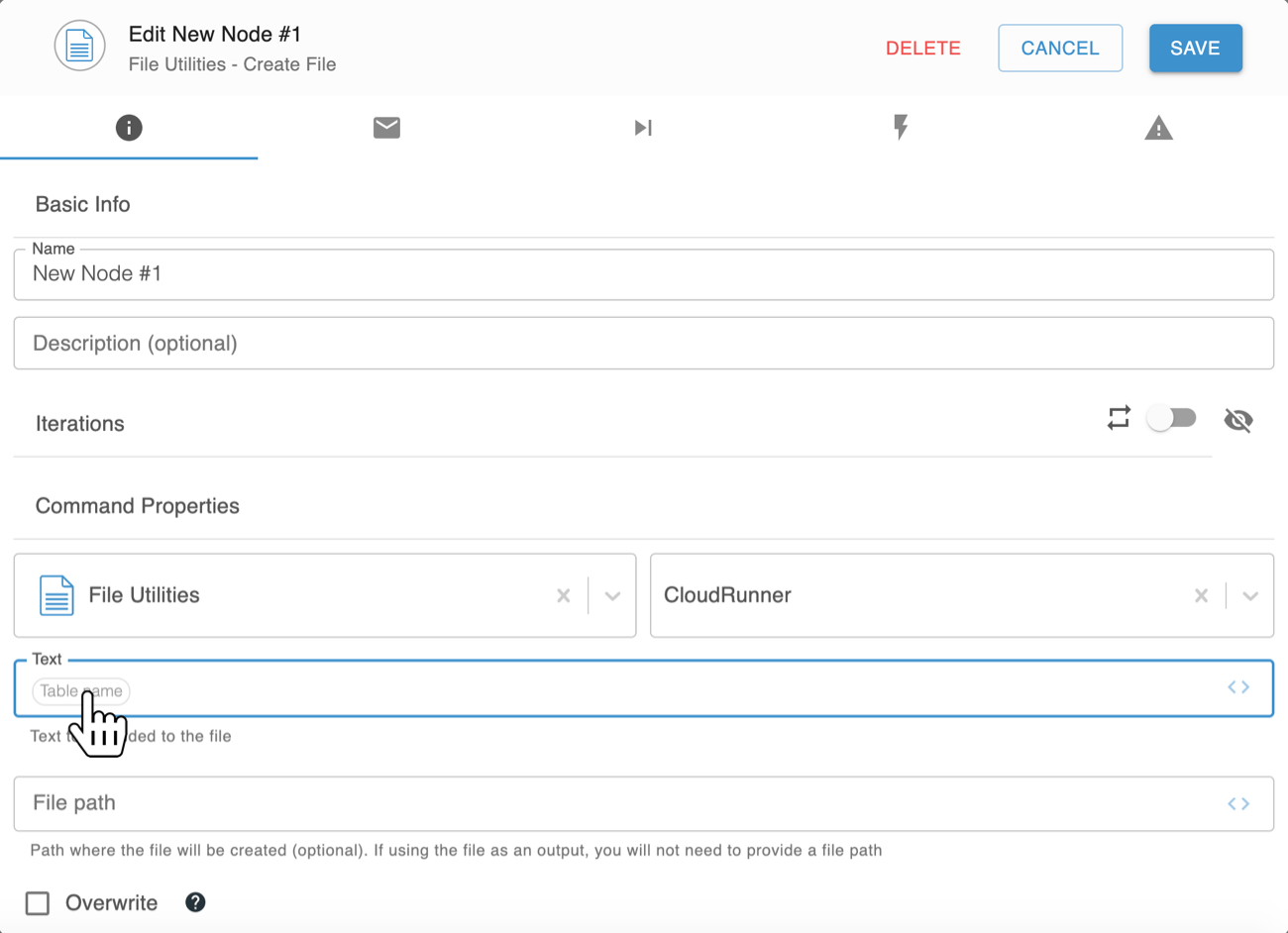The image is a screenshot of a user interface for a software application, likely used for managing or creating nodes within a larger system. At the top of the interface, there is a title that reads "Edit New Node Number One," accompanied by menu options labeled "File," "Utilities," and "Create."

On the right-hand side of the interface, there are three prominent buttons: "Delete," "Cancel," and "Save." Below these buttons, the interface is divided into several sections. The first section is labeled "Basic Info" and contains a text field titled "Name," which is currently filled with "New Node Number One." Directly below this, there is a text field for "Description (optional)."

The next section is titled "Iterations," followed by another section labeled "Command Properties." This section contains options like "File," "Utilities," and "Cloud Runner." 

Within this section, there is a white text box with a blue border around it, making it stand out. The text box is labeled "Text Table Name," and a graphical hand with a pointing finger is depicted, indicating that this is the selected option. The subsequent field is titled "File Path" and includes the instruction: "Path where the file will be created (optional). If using the file as an output, you will not need to provide a file path." 

Finally, underneath this field, there is a checkbox labeled "Overwrite."